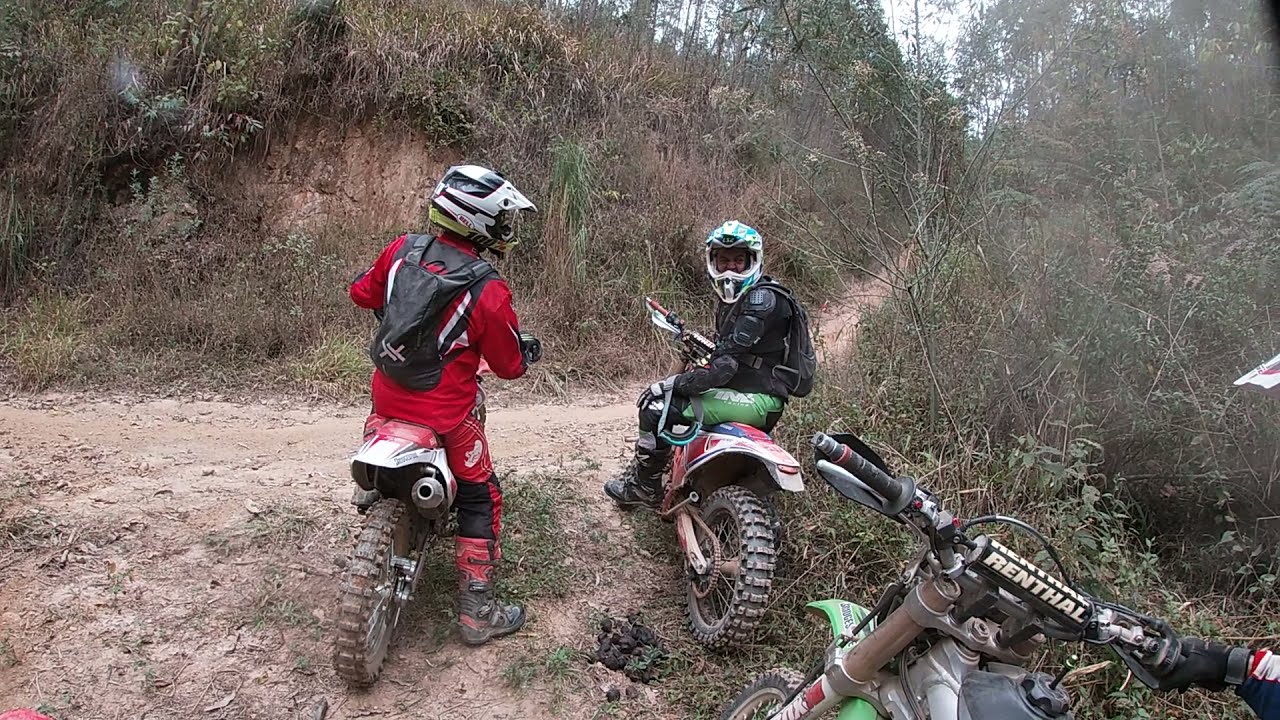Three dirt bikers are poised on their motorcycles along a light brown dirt trail that meanders through verdant vegetation, adorned with tall green and yellow plants on either side. The biker furthest to the right wears a red jumpsuit and a black backpack, his mostly white helmet adorned with black stripes; his motorcycle features a predominantly white rear fender and a mud-splattered back tire. In the center is another rider, clad in a black suit with green pants and carrying a black backpack. His helmet is primarily white with a hint of teal, and his bike also has a dirty back tire, its metal chain visible. The third biker, barely in the frame, only reveals a black-gloved hand gripping the handlebars of a bike with a black cushioning pad in the center emblazoned with "RENTHAL" in uppercase white letters. The trail they are on stretches into the distance, with spots of dirt visible amidst grass and shrubbery, leading towards a hazy, cloud-dotted sky barely peeking through the foliage.